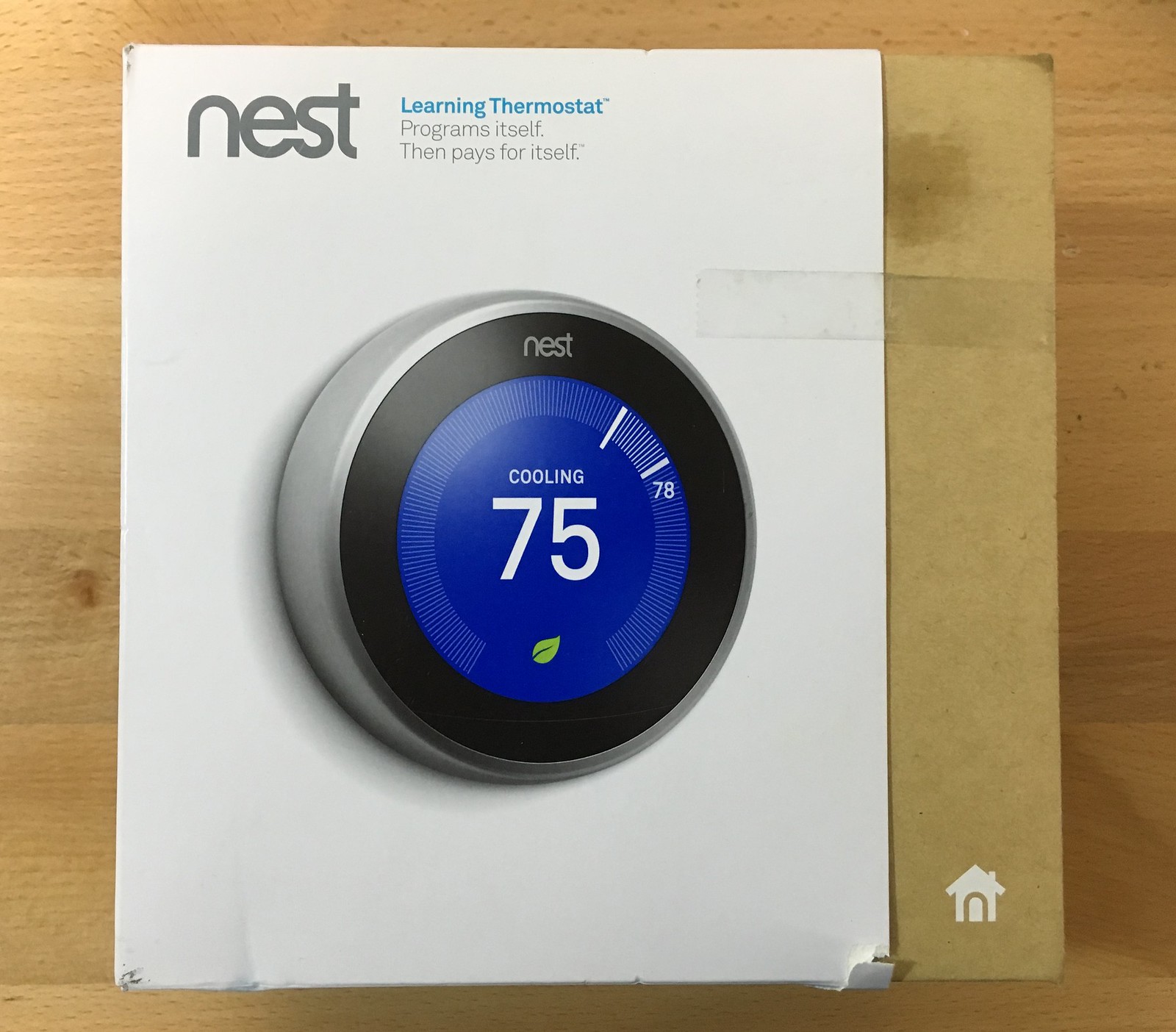The photograph showcases a white square box containing a Nest thermostat. In the top left corner, "nest" is printed in gray letters, followed by "Learning Thermostat" in blue letters. Below that, the phrase "Programs itself. Then pays for itself." is written in gray letters. Dominating the center of the box is an image of the round thermostat, which features a silver outer edge and a black ring on the front face. The display in the center is blue, showing "Cooling 75" in white text. A small green leaf icon appears below the temperature reading, possibly indicating an energy-efficient setting. The display also includes a subtle gauge suggesting various temperature ranges.

The box rests on a light-colored wood surface with visible wood grain, casting a slight shadow to the right. A piece of clear tape secures the box, extending from the white part to a side piece that closely matches the color of the table. In the lower right corner of the box, there is a small computer-generated image of a house.